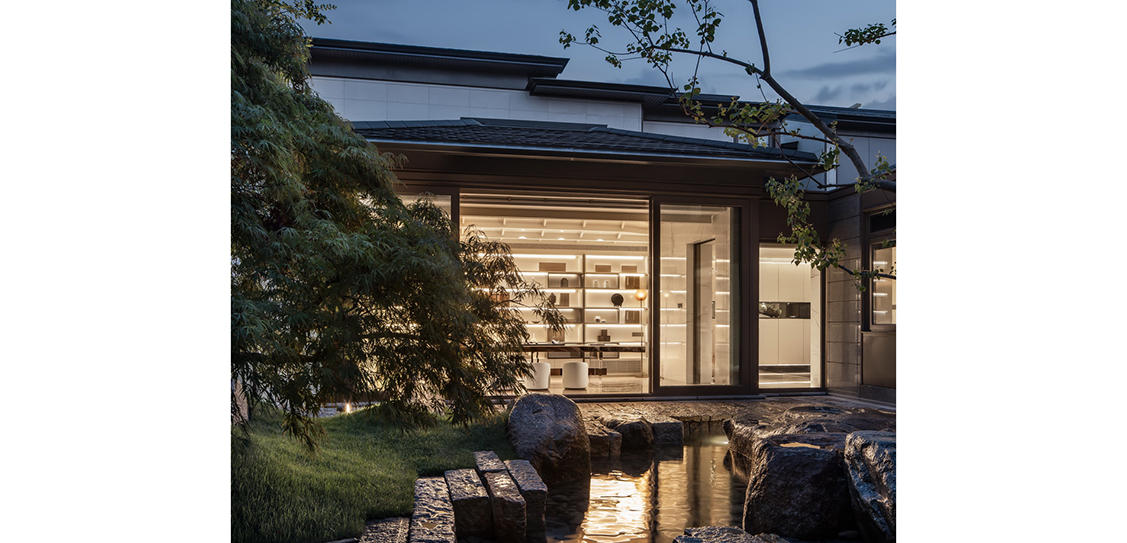This photograph captures the exterior of a contemporary, modern home at dusk, viewed from what appears to be the garden or backyard area. In the foreground, there's a small, man-made pond lined with stones on the right. Just to the left of the pond lies a grassy area with a leafy tree overhanging. The house itself can be seen in the background, characterized by its sleek, minimalist design with clean, straight lines. It features a multi-tiered, low-level roof and large glass windows and doors, allowing a clear view into a bright and well-lit interior. Inside, the house is sparsely furnished, with visible minimalist decor that includes a table, a couple of chairs, and several shelves. The overall ambiance is enhanced by the horizontal lights that illuminate the white, clean interior, creating a stark contrast against the gloomy, dusk sky outside. No people are visible inside or outside the house, emphasizing the serene and immaculate setting.